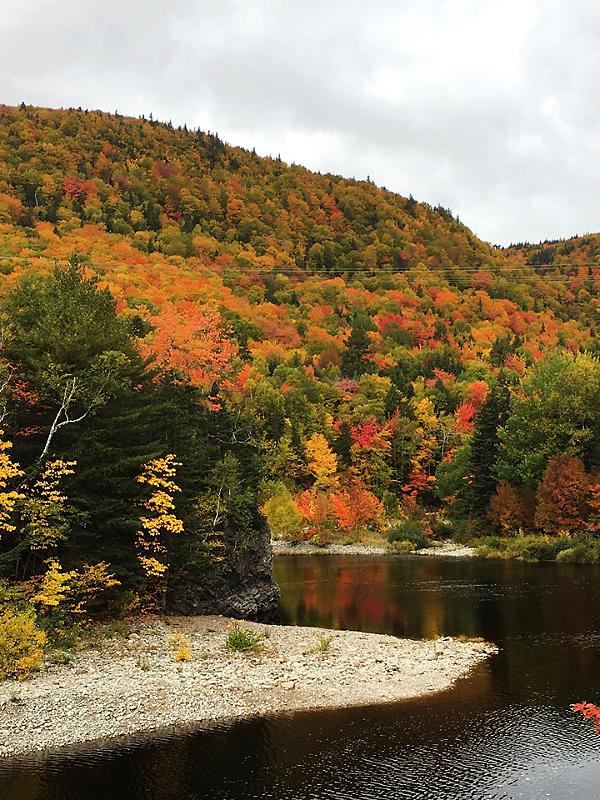The photograph is a detailed landscape scene taken outdoors in broad daylight during autumn. The image captures a sloping hillside densely covered with a variety of trees showcasing vibrant fall foliage in hues of red, yellow, and green. At the base of the hill, a dark grey, almost black lake with subtle ripples is visible. The shoreline is composed of almost whitish sand or gravel, scattered with small rocks, pebbles, and tiny plants or shrubs. The sky above is overcast with gray and white clouds, adding to the overall moody atmosphere of the scene. The setting suggests a forested, wilderness area with thick brush and dense plant life, indicative of the rich and vivid colors typical of the fall season. There is no text overlay on the image.